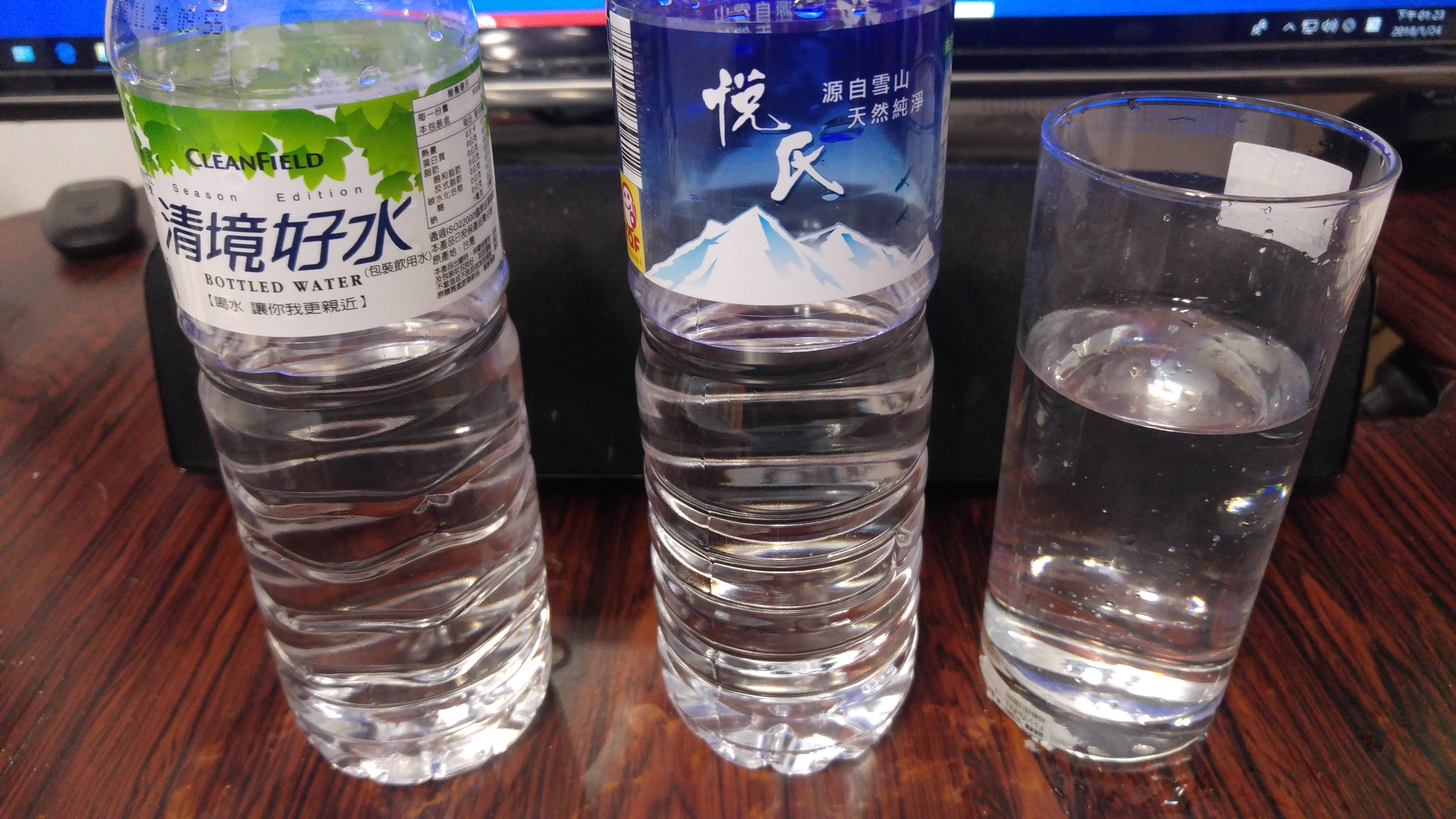The image depicts a dark brown wood grain tabletop interspersed with lighter brown patterns, resembling an office desk. Prominently situated on the desk are two plastic water bottles and a glass of water. The bottle on the left displays the brand "CLEANFIELD" with a white label featuring blue highlights, alongside Japanese characters that translate to "Season Edition." The bottle is half-full. Positioned beside it, another half-full plastic bottle showcases Japanese text and a blue logo with an outline of a mountain topped with blue and white snowcaps.

To the right of these bottles stands a glass of water, filled slightly more than halfway. Dominating the background is a computer monitor displaying a Windows toolbar, though specifics like the time are unclear. Nearby, a black bag rests in front of the monitor, accompanied by what appears to be a remote control or key fob.